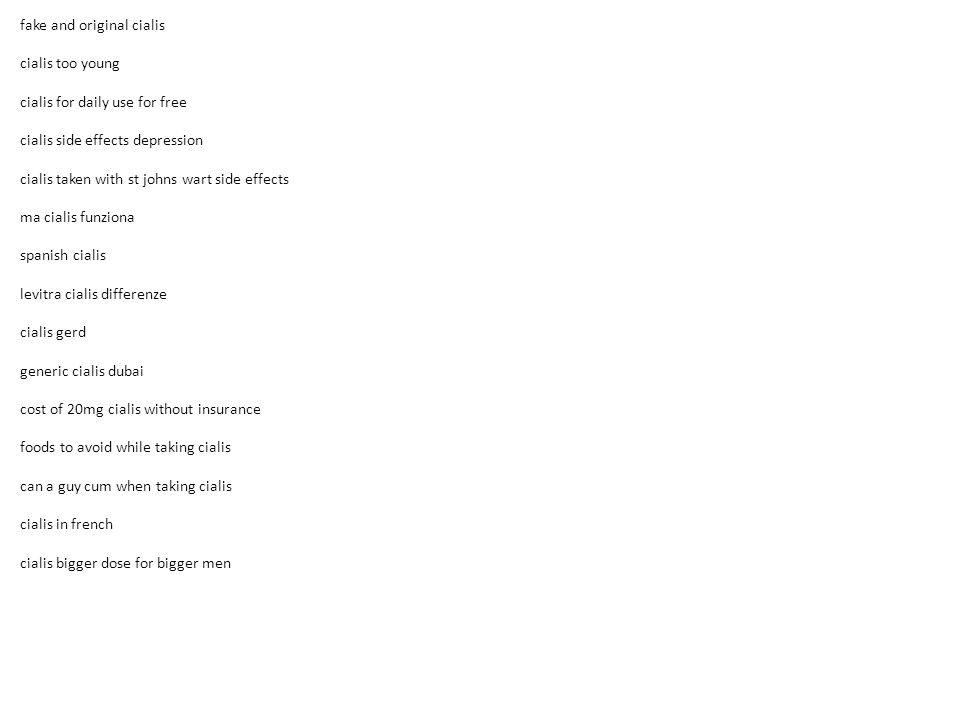A left-aligned list of small black print text occupies the left half of the image, while the right half remains blank and white. The list is neatly organized, with each entry separated by a space. The text at the top of the list reads various phrases, starting with "fake and original Cialis" and continuing with topics such as "Cialis too young," "Cialis for daily use for free," "Cialis side effects depression," "Cialis taken with St. John's wort side effects," "Ma Cialis Funzona," "Spanish Cialis," "Levitra Cialis Difference" (with "Difference" misspelled as "D-I-F-F-E-R-E-N-Z-E"), "Cialis GERD," "generic Cialis Dubai," "cost of 20 milligrams Cialis without insurance," "food to avoid while taking Cialis," "can a guy come when taking Cialis," "Cialis in French," and concluding with "Cialis bigger dose for bigger men."